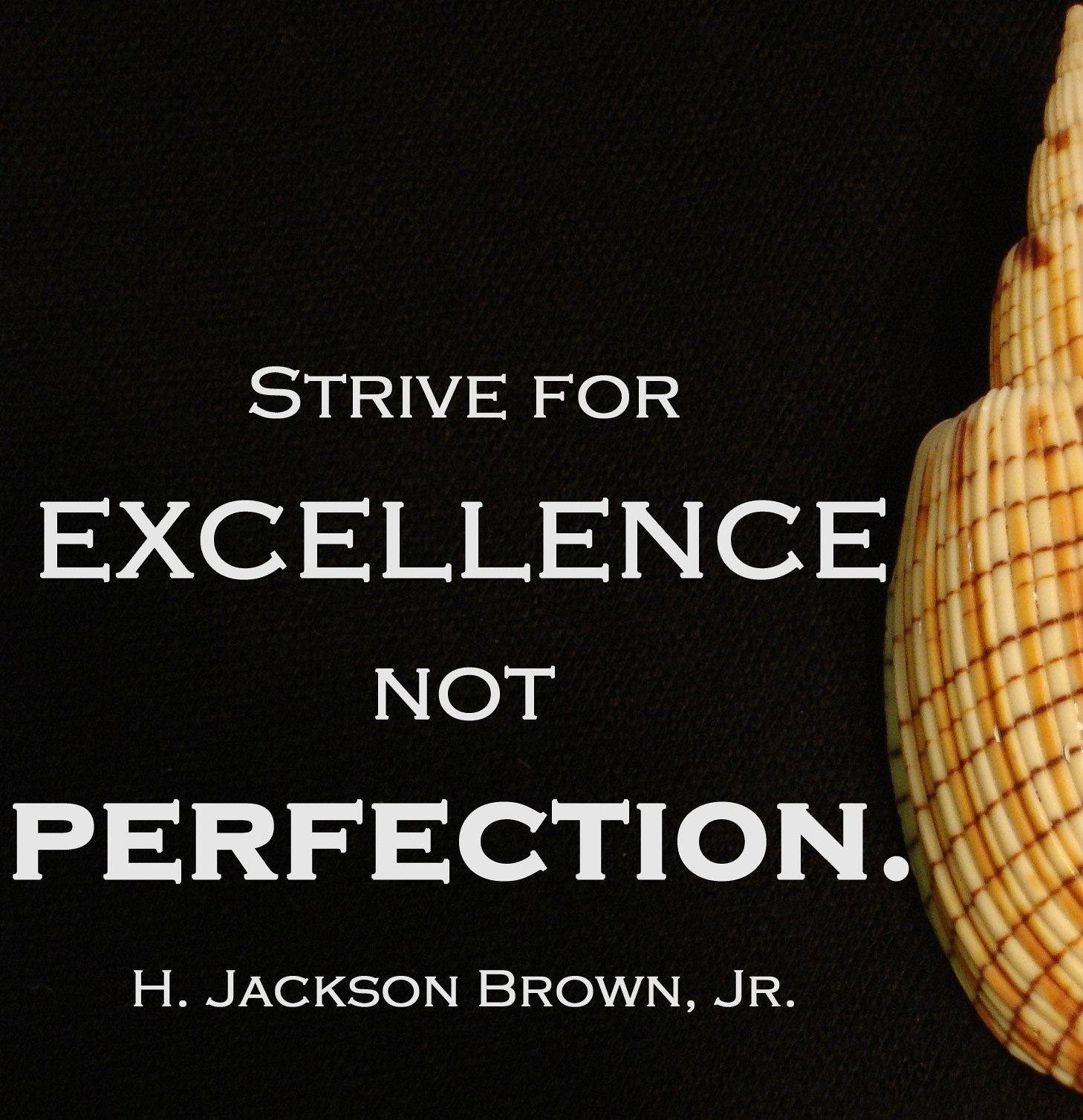The image features a sign against a black background, with no people present. The background appears to have a cloth-like texture. On the right side of the image, there is a partially visible object that resembles a seashell in cream color with brown horizontal stripes. This object tapers off as it extends upward. The focus of the image is the text, which is centered but slightly shifted to the left to accommodate the seashell. The white lettering reads, "Strive for excellence, not perfection," attributed to H. Jackson Brown Jr., also in white text at the bottom. The purpose of the image is ambiguous; it could be a cover for a magazine, an advertisement, or part of a project.